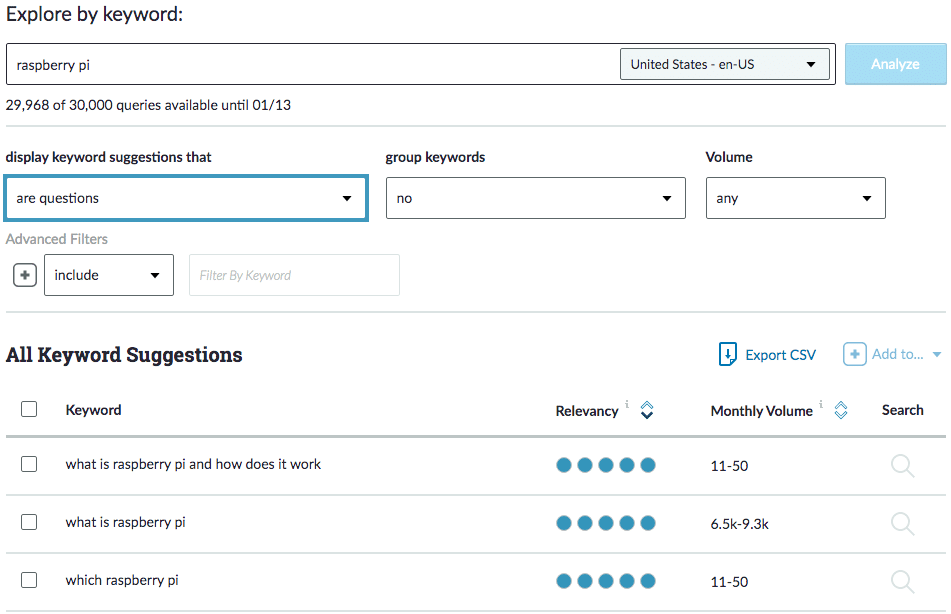The image displays an interface for a keyword analysis tool. At the top, the screen features a prompt titled "Explore by Keyword," accompanied by a search bar where "United States" is initially set as the default search location but can be adjusted via a dropdown menu. The current search query is "Raspberry Pi." A prominent blue button labeled "Analyze" is visible.

Below this section, the screen shows usage statistics indicating that 29,968 out of 30,000 queries are available until January 13th. The keyword suggestion section beneath contains various elements. It features a tab for questions and grouped keywords, with an option to filter by those with no search volume. Advanced filters are also present, with an "Include" dropdown menu that is currently empty.

Users can export the keyword suggestions to a CSV file or add them to a list via a dropdown menu. The first keyword suggestion is "What is Raspberry Pi?" with a relevancy rating of 5 out of 5 and a monthly search volume between 11 and 50, accompanied by a search button. The second suggestion, also highly relevant with a 5 out of 5 rating, reads "What is Raspberry Pi again?" with an estimated search volume ranging from 600.9K to 9K. The final suggestion is "Which Raspberry Pi," similarly rated at 5 out of 5 with a monthly search volume between 11 and 50.